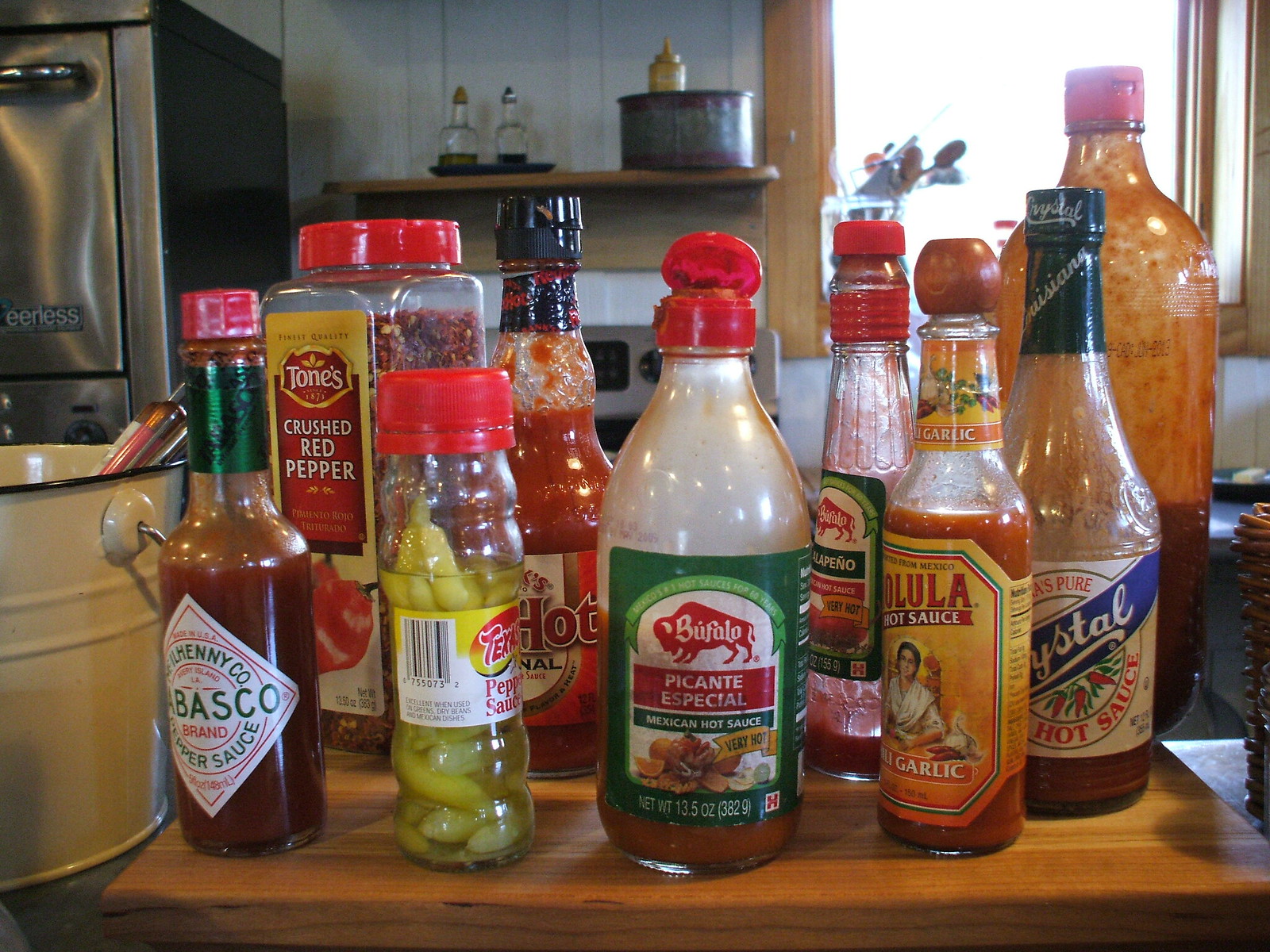The image is a detailed, color photograph taken inside a kitchen, centered on a wooden countertop. Arranged on a brown wooden cutting board atop the countertop are approximately ten bottles of various hot sauces, each with different shapes and labels. Among the identifiable sauces are Tabasco, Mexican hot sauce, picante especial, garlic hot sauce, crushed red pepper, and pepperoncinis. Notable labels include "Buffalo," "Crystal" with a distinctive blue strip, and several bottles with red lids. In the background, there is a stainless steel stove with control knobs visible, a stainless steel wall oven to the left, and a white pot underneath. A window on the top right of the image allows white light to stream through, adding to the kitchen setting.